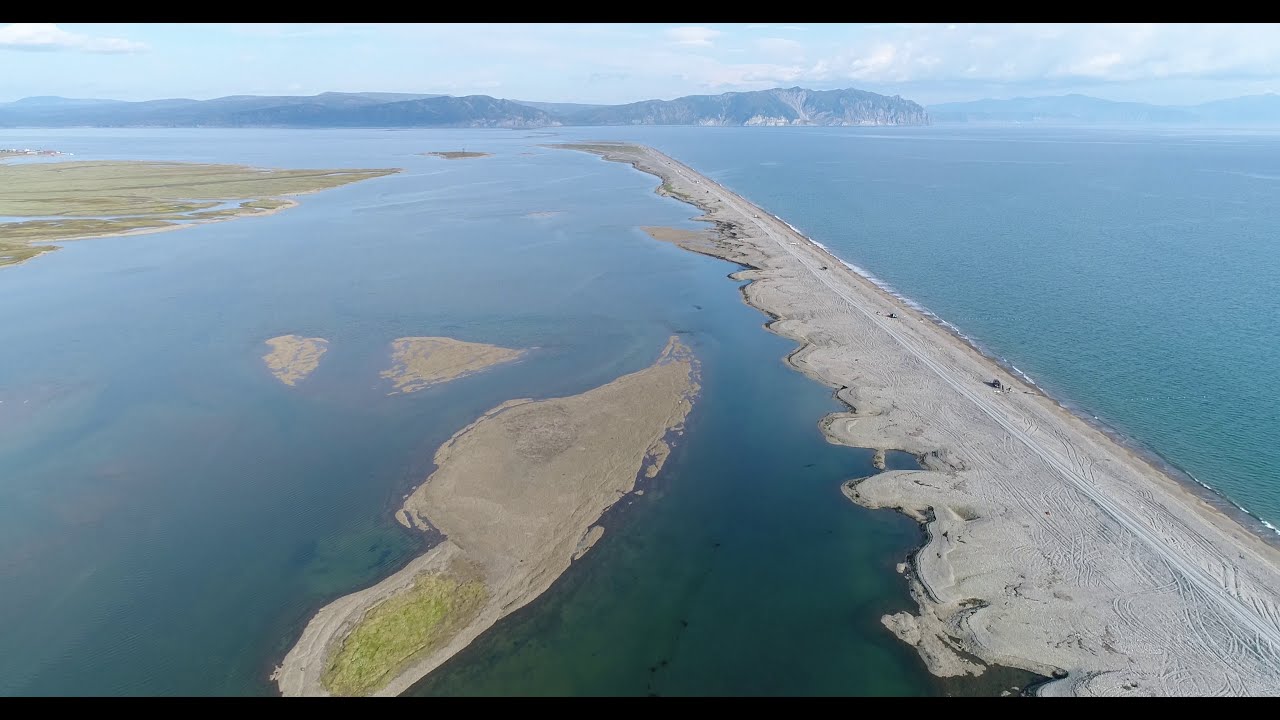This landscape image captures a stunning outdoor scene from an aerial perspective. Framed by two black banners at the top and bottom, the viewer is presented with a vast body of vibrant blue water. A slender, possibly sandbar-like landmass stretches almost to the horizon, flanked by smaller islets to the left. The narrow landmass appears unpaved with visible tire marks, hinting at off-road vehicle use, and scattered people can be seen on it. Along the shorelines of these landmasses, patches of green vegetation, likely moss or grass, contrast against the predominantly grey and tan, clay-like terrain. In the background, a mountain range partially shrouded by cloud coverage extends across the horizon, its rocky features interspersed with dark-hued trees or bushes. The sky above is a mix of light and deep blue, accentuated by white clouds, encapsulating the natural beauty of the scene.